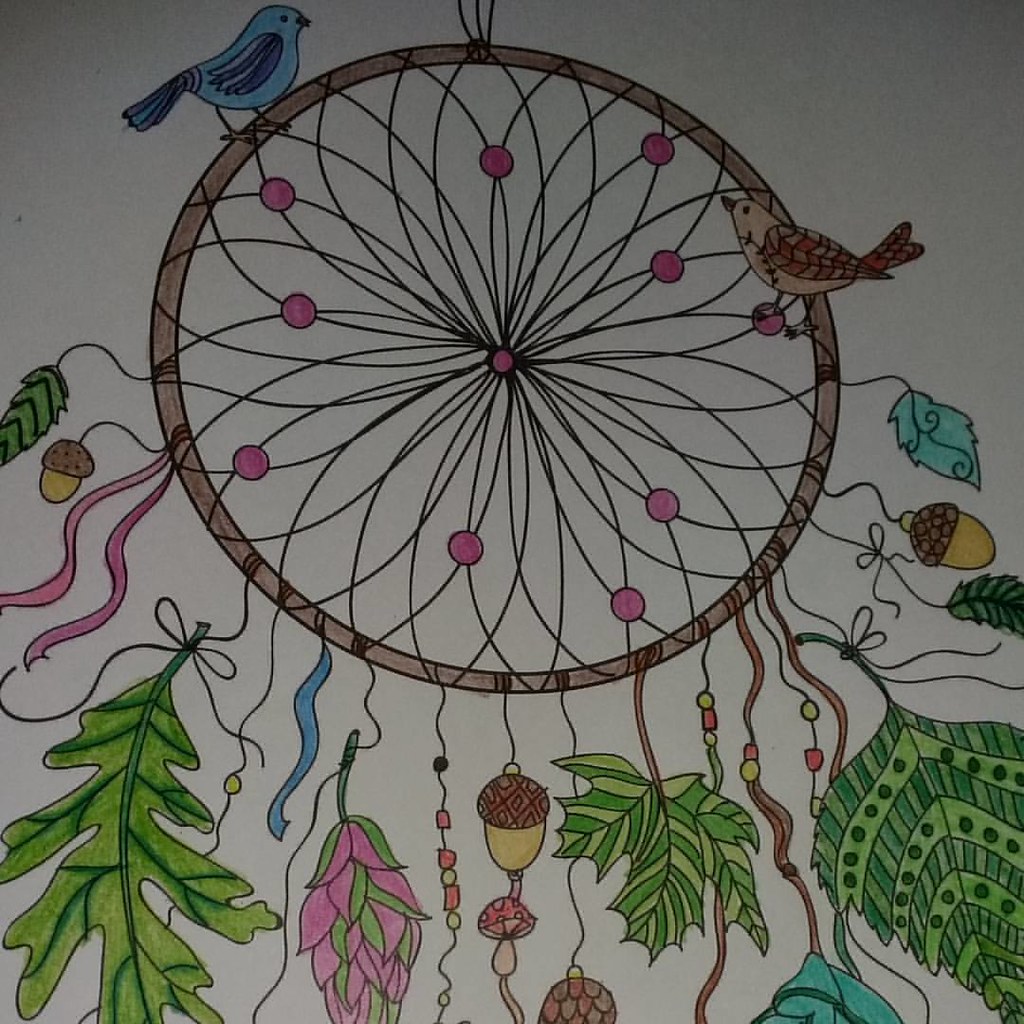This intricate drawing evokes the charm and detail of an adult coloring book page, featuring a meticulously colored black line illustration on a light gray background. Central to the image is a circular, brown decorative element resembling a wind chime, though it lacks any actual chimes. Inside the circle, delicate wires crisscross to form a floral pattern, accentuated by dark pink circles along the outer lines.

Perched on the circle are two vibrantly hued birds: one at the top left, colored in shades of blue, and another at the top right, adorned in tan and brown. From the bottom of this circular centerpiece dangle a series of detailed elements, beginning with a leaf on the far left, followed by an acorn, pink ribbons, a larger green oak leaf, a light blue ribbon, a flower top, another acorn, a mushroom, a pine cone, more leaves interspersed with various ribbons and beads, culminating in yet another series of green leaves and acorns. The attention to detail in each element showcases the artist's patience and creativity, making this piece a true feast for the eyes.